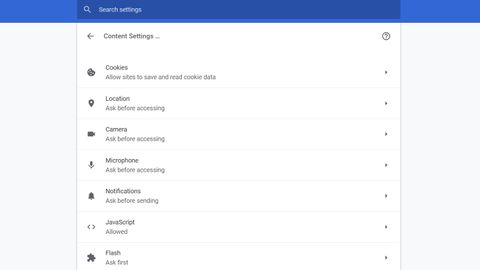The screenshot captures a browser settings page with a detailed top section and various settings listed below. At the top, a blue bar spans from left to right, with a darker center featuring a white magnifying glass icon followed by the text "Search settings." Below, on a white background with gray borders, there's a left-facing arrow labeled "Content settings" and a circled question mark to the right.

The subsequent section lists different settings, each with an associated icon and text: 

1. A cookie icon next to "Cookies," followed by "Allow sites to save and read cookie data."
2. A pin icon next to "Location," followed by "Ask before accessing."
3. A video camera icon next to "Camera," followed by "Ask before accessing."
4. A microphone icon next to "Microphone," followed by "Ask before accessing."
5. A bell icon next to "Notifications," followed by "Ask before sending."
6. Open and close brackets next to "JavaScript," denoted as "Allowed."
7. A puzzle piece icon next to "Flash," followed by "Ask first."

Each setting to the right features a small circular button or arrow, though the exact symbol is unclear due to the small font size.